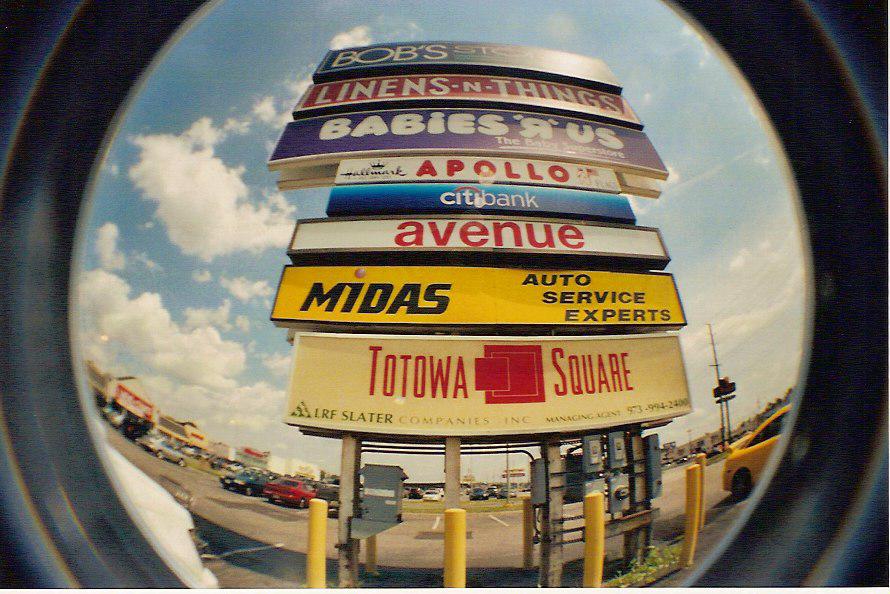In this high-quality photograph taken through a fisheye lens, we see a large, convex image of a prominent strip mall sign standing in a spacious parking lot under a blue sky with scattered clouds. The fisheye effect creates a circular, curved vignette, cropping some details at the edges and enhancing the curvature of the scene. At the top of the sign, barely legible due to sunlight glare, is "Bob's". Below it, signs for various stores are stacked vertically, readable as: "Linens and Things" in red, "Babies R Us" in blue, "Hallmark Apollo" in white, "Citibank" in blue, "Avenue" in white with red text, "Midas Auto Service Experts" in yellow, and "Tatawa Square" in white. Surrounding the sign are concrete bollards for protection. The parking lot is filled with a mix of cars in yellow, red, blue, and more, and a delivery truck is seen near the base of the sign. In the distance, other stores and businesses are visible, suggesting a busy commercial area.